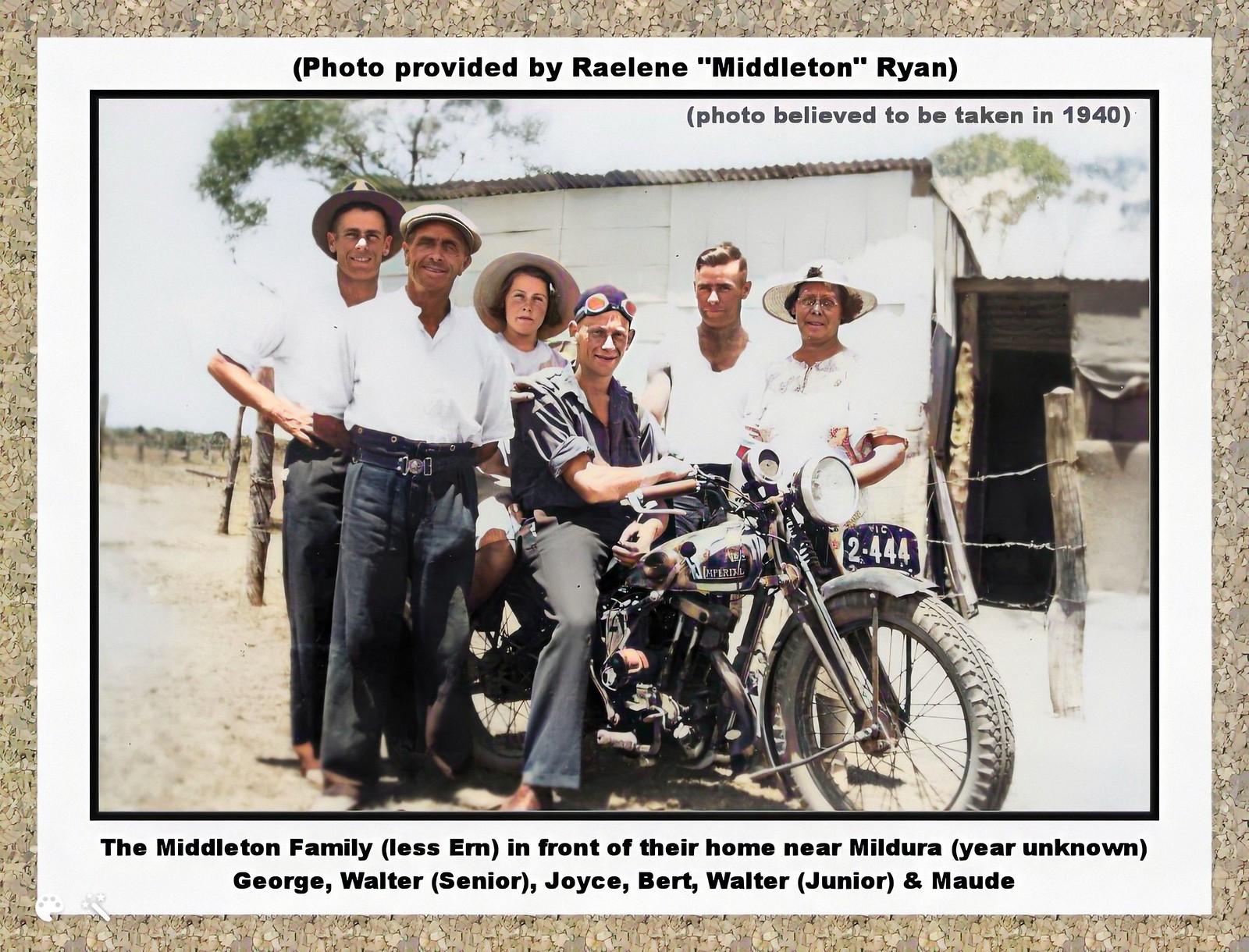This photograph, believed to have been taken in 1940, depicts a man dressed in dark clothes and goggles seated on a motorcycle in the center. To his left stand two men and a woman, while to his right are another man and woman. The group is outside, with the backdrop of a small house and trees, suggesting a rural setting near Mildura. All individuals except the young man on the motorcycle wear short-sleeved white shirts; some are barefoot, and the women are wearing hats. At the top of the image, a note reads "Photo provided by Raylene Middleton Ryan." Below the photo, in black font, it states: "The Middleton family, Les Earn, in front of their home near Mildura, year unknown." The names listed are George, Walter Sr., Joyce, Burt, Walter Jr., and Maude. The photograph is framed by a white border with additional text and an outer gray stone-like border.